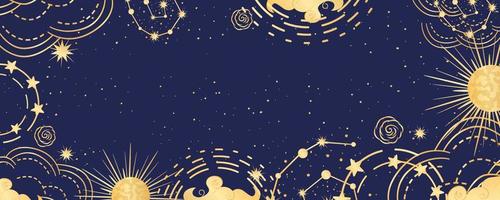This horizontal rectangular image portrays a stylized drawing of the night sky with a deep navy, nearly black background scattered with small white spots symbolizing stars. Dominantly featured on the right center of the image is a gold-colored celestial body that resembles a moon with crater markings, yet it also emanates thin rays reminiscent of a sun. The borders of the image are adorned with intricate celestial designs in a golden hue, including swirls, spirals, and cloud-like patterns that suggest constellations and other astronomical elements. Another sun-like figure appears in the lower left corner, enhancing the cosmic theme. Overall, the drawing emphasizes an enchanting, cartoon-like portrayal of outer space, featuring aspects of both the night sky and celestial bodies.